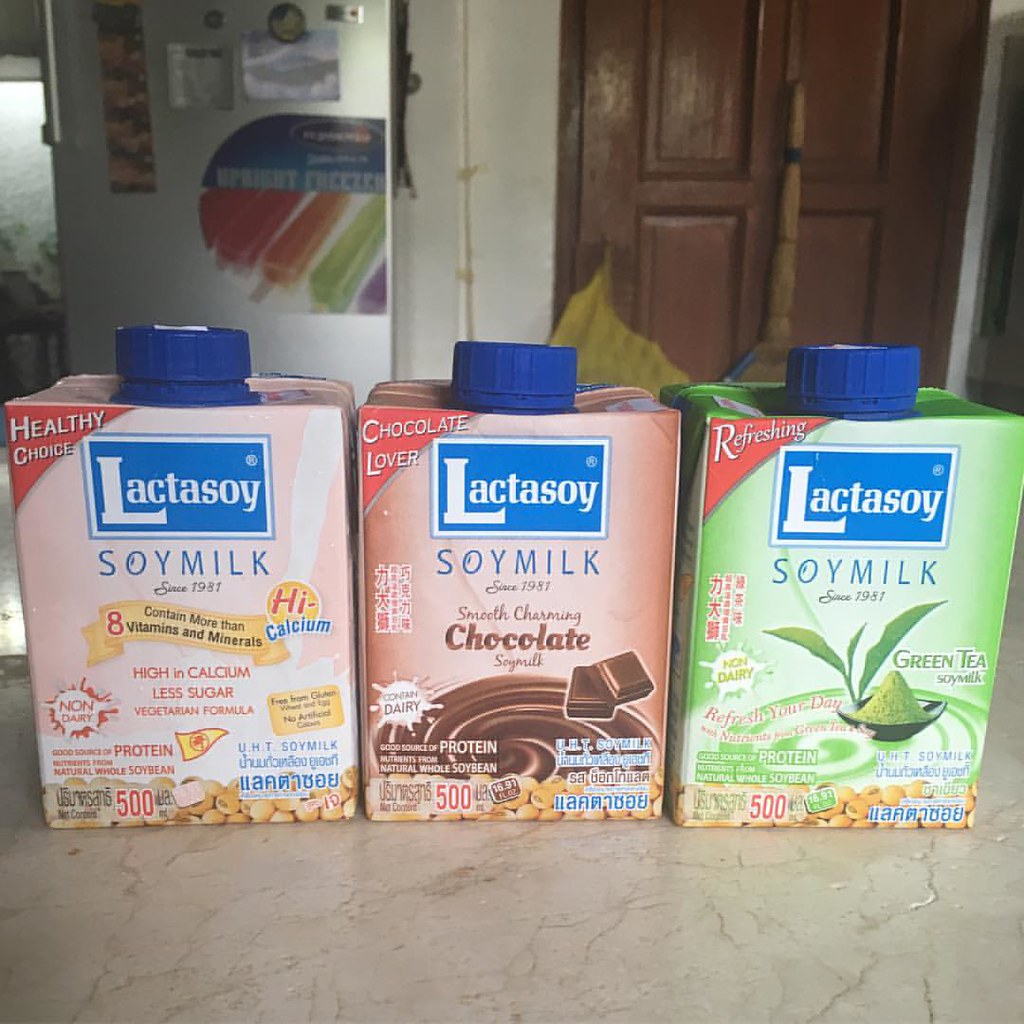This image showcases three upright Lactasoy soy milk boxes on a tan marble countertop, each with a dark blue plastic cap. The boxes are labeled with the brand's dark blue and white logo followed by "Soy Milk" and "Since 1981." From left to right, the flavors are "Healthy Choice," "Chocolate Lover," and "Refreshing Green Tea." The "Healthy Choice" box emphasizes high calcium, eight vitamins and minerals, and a vegetarian formula, with a non-dairy sticker near the bottom. The "Chocolate Lover" box features smooth, charming chocolate soy milk, and imagery of chocolate pieces. The "Refreshing" box features green tea soy milk with illustrations of green tea leaves and a green squirrel. In the background, a silver metallic door with a colorful poster of popsicles is on the left, beside a dark brown wooden door.